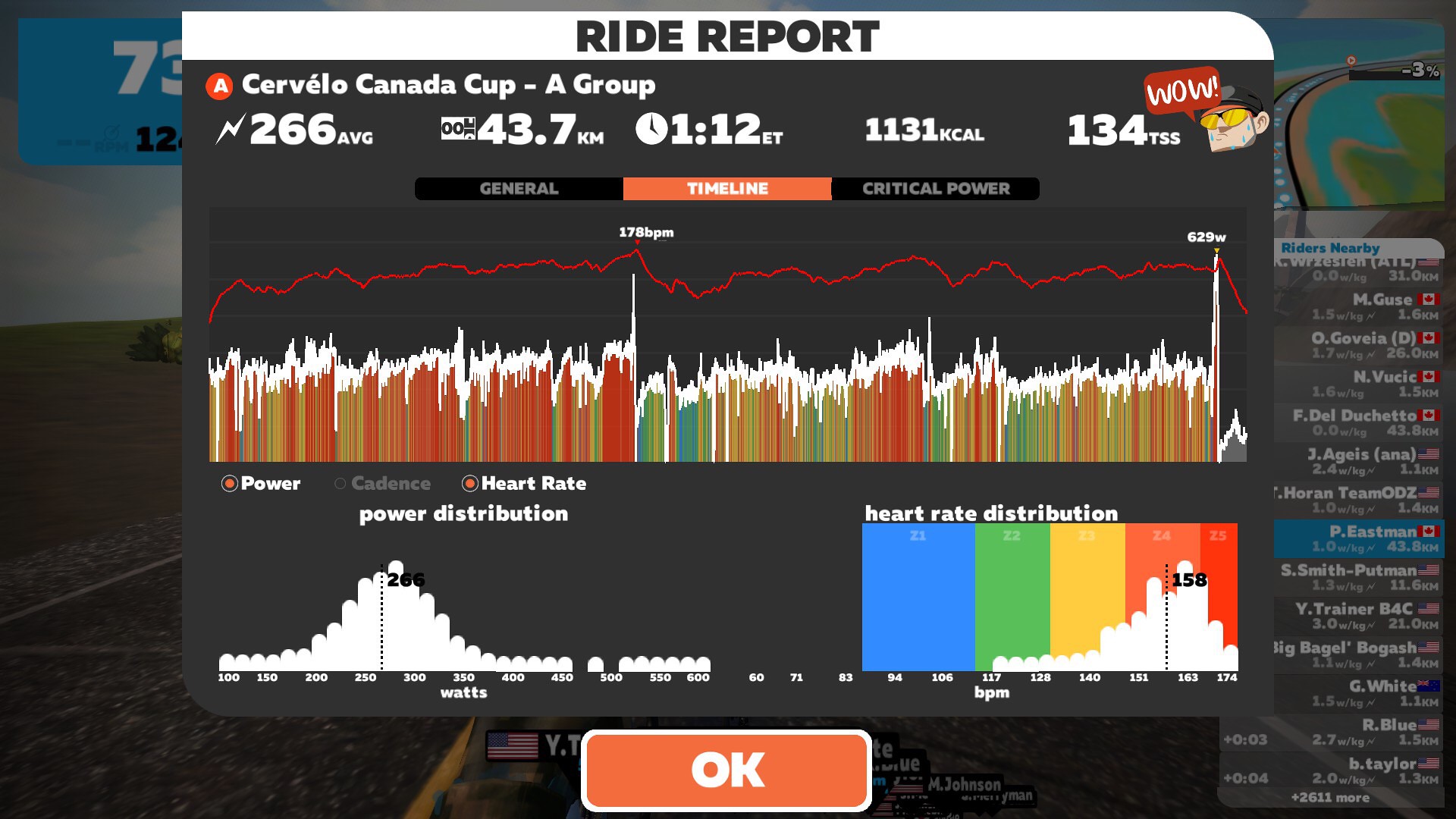This high-definition image, seemingly a computer or television screenshot, showcases a detailed Ride Report for the Cervelo Canada Cup Dash A Group. The dark, black background accentuates the colorful bar graphs and line charts in red, gold, green, and white. At the top, "Ride Report" is prominently displayed in black lettering on a white border, immediately followed by performance metrics: average speed of 43.7 km/h, distance of 266 km, elapsed time (ET), 1131 kcal burned, and a Training Stress Score (TSS) of 134. A small cartoon drawing of a man in a black cap and yellow sunglasses exclaims "Wow" in a white and red speech bubble next to these numbers. Below the metrics, tabs labeled "General," "Timeline," and "Critical Power" are visible, along with a detailed chart indicating heart rate peaks at 178 BPM and power cadence metrics. Lower segments of the image feature smaller bar graphs, including one titled "Heart Rate Distribution" in rainbow colors, and an orange button labeled "OK" bordered in white, suggesting an interactive element. The image likely represents either a real-time performance monitoring interface or a post-ride analysis report.